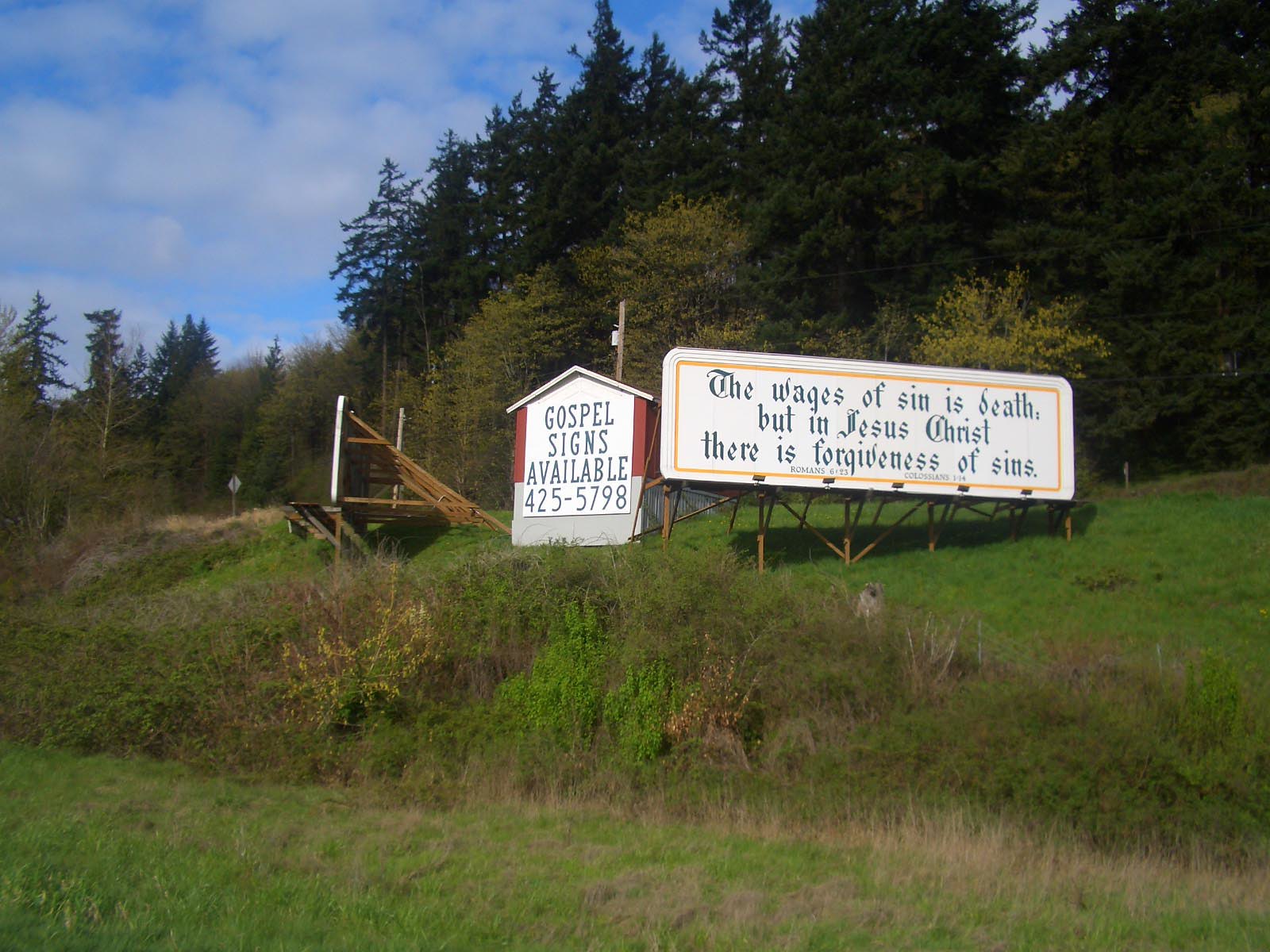The image showcases a picturesque countryside scene featuring a set of two distinct signs. In the foreground, the lush, bright green grass of a mountainside contrasts with the dense layers of dark and light green trees in the background, forming a thick forest under a clear blue sky with scattered clouds. On the left, a small, red brick shed catches the eye, adorned with a white-painted sign that reads, "Gospel Signs Available" along with the phone number "425-5798" in black letters. The shed is situated next to a larger, white billboard with Gothic serif font outlined in yellow, conveying the solemn message, "The wages of sin is death, but in Jesus Christ, there is forgiveness of sins." The billboard is illuminated by ground lights, indicating it is visible both day and night. Together, the elements create a serene yet thought-provoking countryside tableau that merges natural beauty with a spiritual reminder.